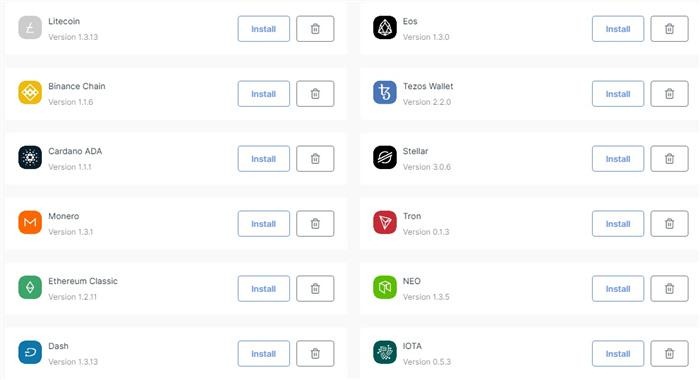The image depicts an application store with a white background. There are two prominent columns displaying various applications that can be installed or deleted. Each column contains six applications. Beneath each application, its version is listed. Additionally, there is a blue "Install" button and a gray trash can icon for deletion.

In the left column, starting from the top, we have:

1. Litecoin
2. Viance
3. Binance Chain
4. Cardano (ADA)
5. Monero
6. Ethereum Classic

In the right column, from the top, we have:

1. EOS
2. Tezos Wallet
3. Stellar
4. Tron
5. Neo
6. IOTA